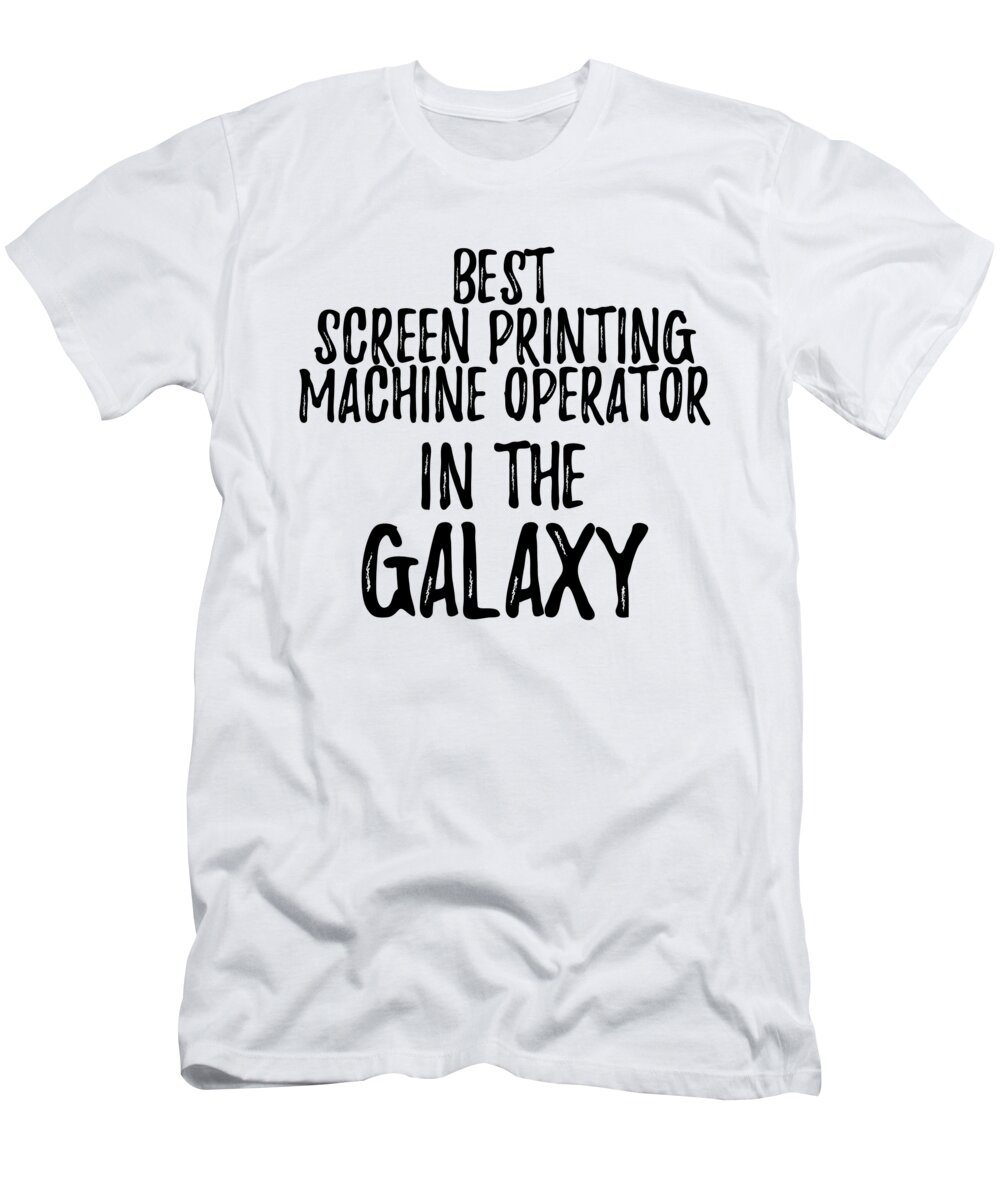The image features a white t-shirt centered against a pure white background, suggesting it has been isolated using Photoshop. The t-shirt, which appears to be slightly crinkled and un-ironed, seems to be a men's shirt as it lacks curves typical of women's apparel and looks a bit larger than average. The shirt boasts bold, black text in an informal sans serif font, mimicking handwritten magic marker style but clearly digitally created due to the identical repetition of letters. The text on the shirt reads, "BEST SCREEN PRINTING MACHINE OPERATOR IN THE GALAXY," spread out over five lines with "GALAXY" in a larger font size than the rest. Shadows under the shirt enhance the wrinkled effect, and the collar appears slightly small, adding to the impression of a custom-made item for a specific individual.